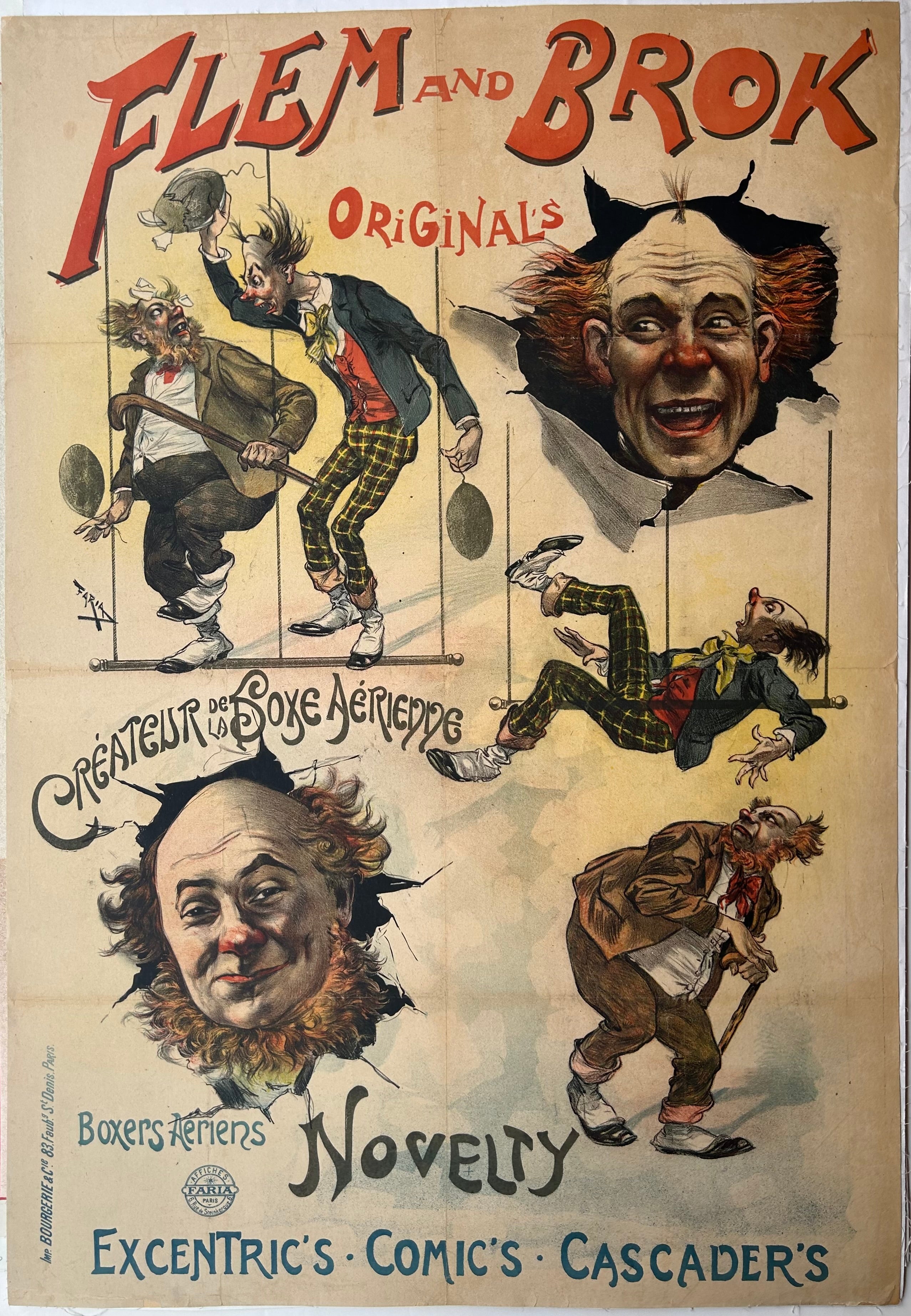This vintage advertisement features the comedic duo "Flem and Brock Originals" showcased in a series of intricate caricature illustrations. Dominating the top of the image, the duo's name is prominently displayed in bold red font. The upper left corner presents two clowns, with a tall, skinny clown standing behind a shorter, rotund one, raising his left arm with an object aloft, as the shorter clown glances back over his shoulder. 

In the upper right corner, a clown with a bald head, red nose, and wild red-orange hair appears to be bursting through a crumbling wall. Beneath him, another clown dangles precariously from a trapeze bar. The lower left corner is marked with the phrase "Creature de la Foxcarion" and features another bald-headed, red-nosed clown, similarly breaking through a disintegrating wall—perhaps hinting at a recurring theme.

The final depiction, in the lower right corner, shows a clown using a cane, looking back over his shoulder. At the bottom of the image, the words "Novelty, Eccentrics, Comics, Cascaders" are inscribed, further emphasizing the eclectic and whimsical nature of the content. This vividly detailed illustration, likely from the 1920s or 30s, captures the essence of classic clowning, complete with playful antics and exaggerated personalities, set against a backdrop of vintage charm.